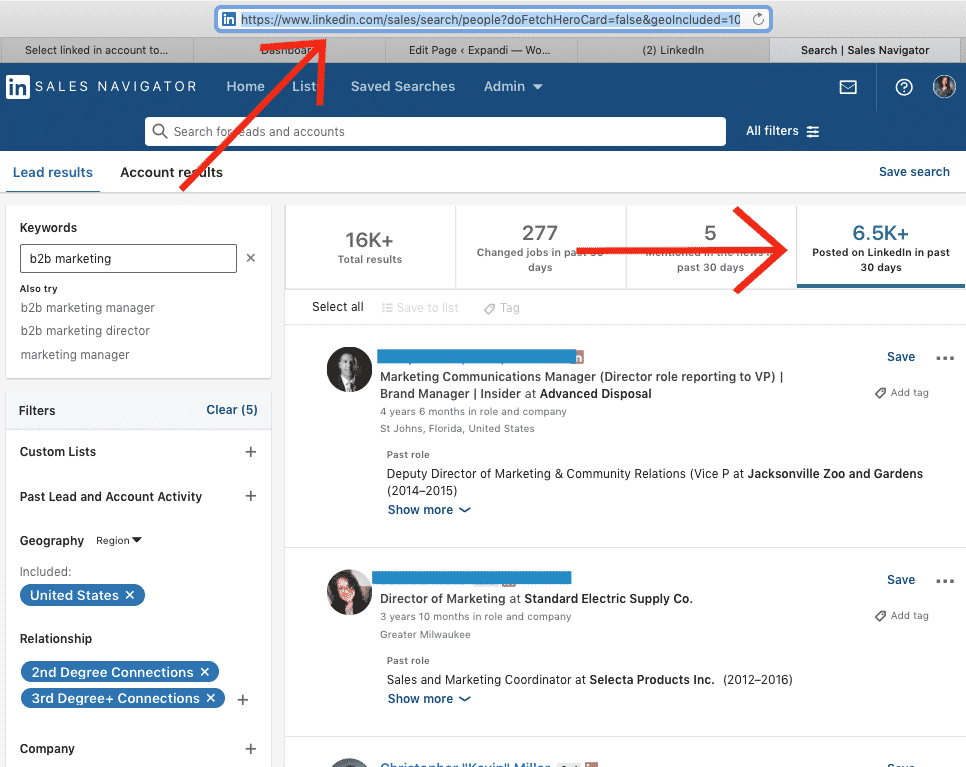The image depicts a screenshot of a LinkedIn Sales Navigator page. At the top, there is a prominent long blue navigation bar, highlighted in light blue, featuring the URL "www.linkedin.com/sales/search/people." Below this, the background shifts to gray, where several interface options are visible starting from the left: a prompt to "Select LinkedIn account 2," followed by "Edit page (2)" and "Search Sales Navigator."

Further below, the background turns to navy blue, displaying the LinkedIn logo (the letters "IN" in white within a square) next to the text "Sales Navigator." Moving downward, the image shows two categories: "Lead Results" and "Account Results," with a red arrow pointing upwards to the URL bar at the top of the screen.

To the right, another red arrow originates next to the text "277 changed jobs," extending to and highlighting "6.5k+ posted on LinkedIn in the past 30 days." Finally, the lower section includes two profile pictures in circular frames: the first, in black and white, is of a man in a suit, while the second, below, is a colored image of a woman wearing glasses with dark brown hair.